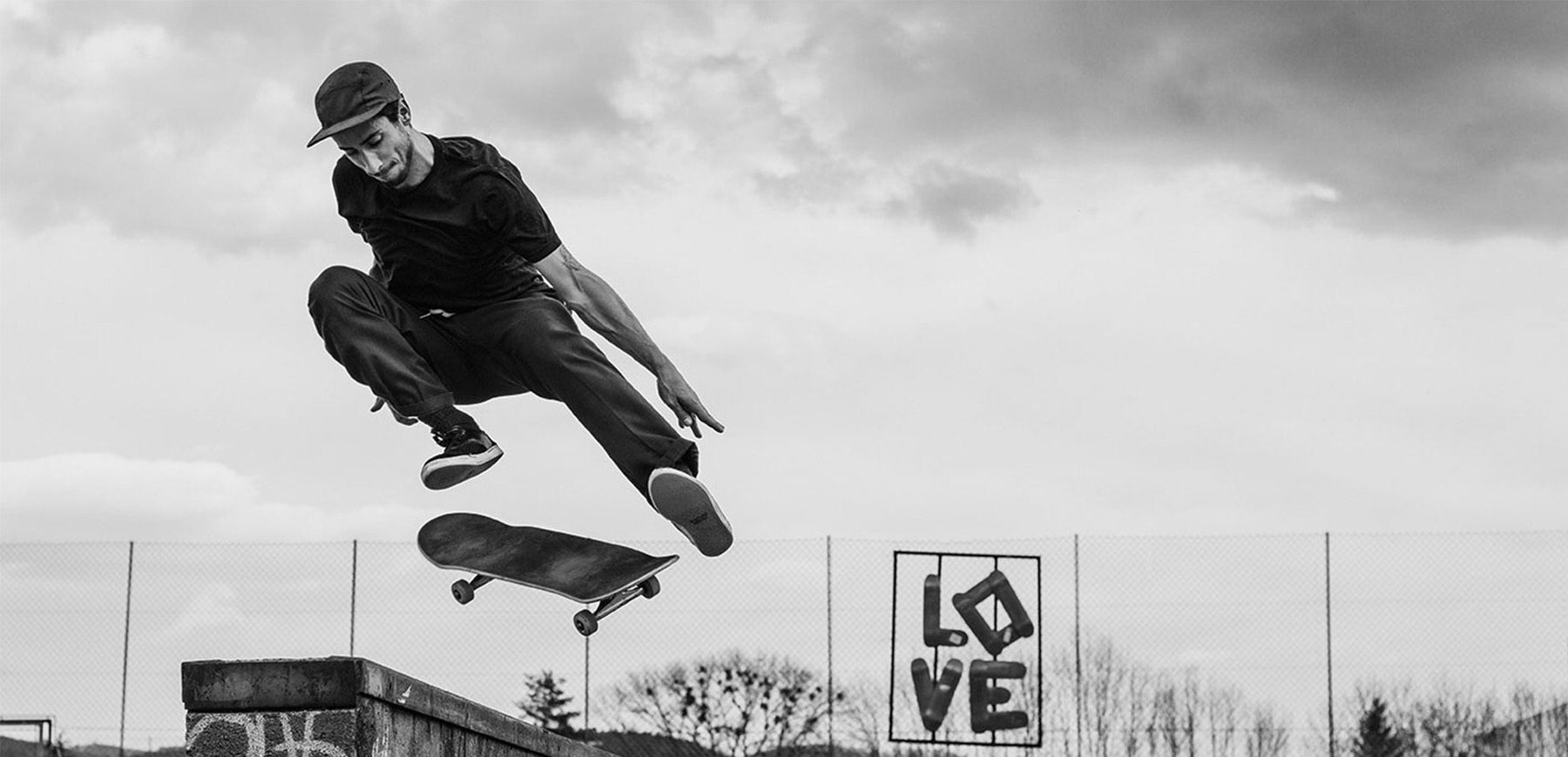In this black and white photograph, a skateboarder is captured midair during an impressive jump, positioned on the left-hand third of the image. His body forms a dynamic figure with his right knee bent upward, his left leg extended parallel to his outstretched arm, and his skateboard even with him but without any contact. The skater is wearing a dark baseball cap, dark t-shirt, dark jeans, and dark sneakers, all in stark contrast to the lighter background. Below him, a concrete pedestal or wall marked with white graffiti stands, suggesting he is executing a trick over it. The backdrop features a chain-link fence adorned with the word "LOVE," creatively spelled out using old skateboard decks. The sky is overcast and largely white, creating a somber tone that emphasizes the gray clouds overhead. Low, sparse trees with what appears to be birds contribute to the composition, inferring a scene set in a desolate urban environment.